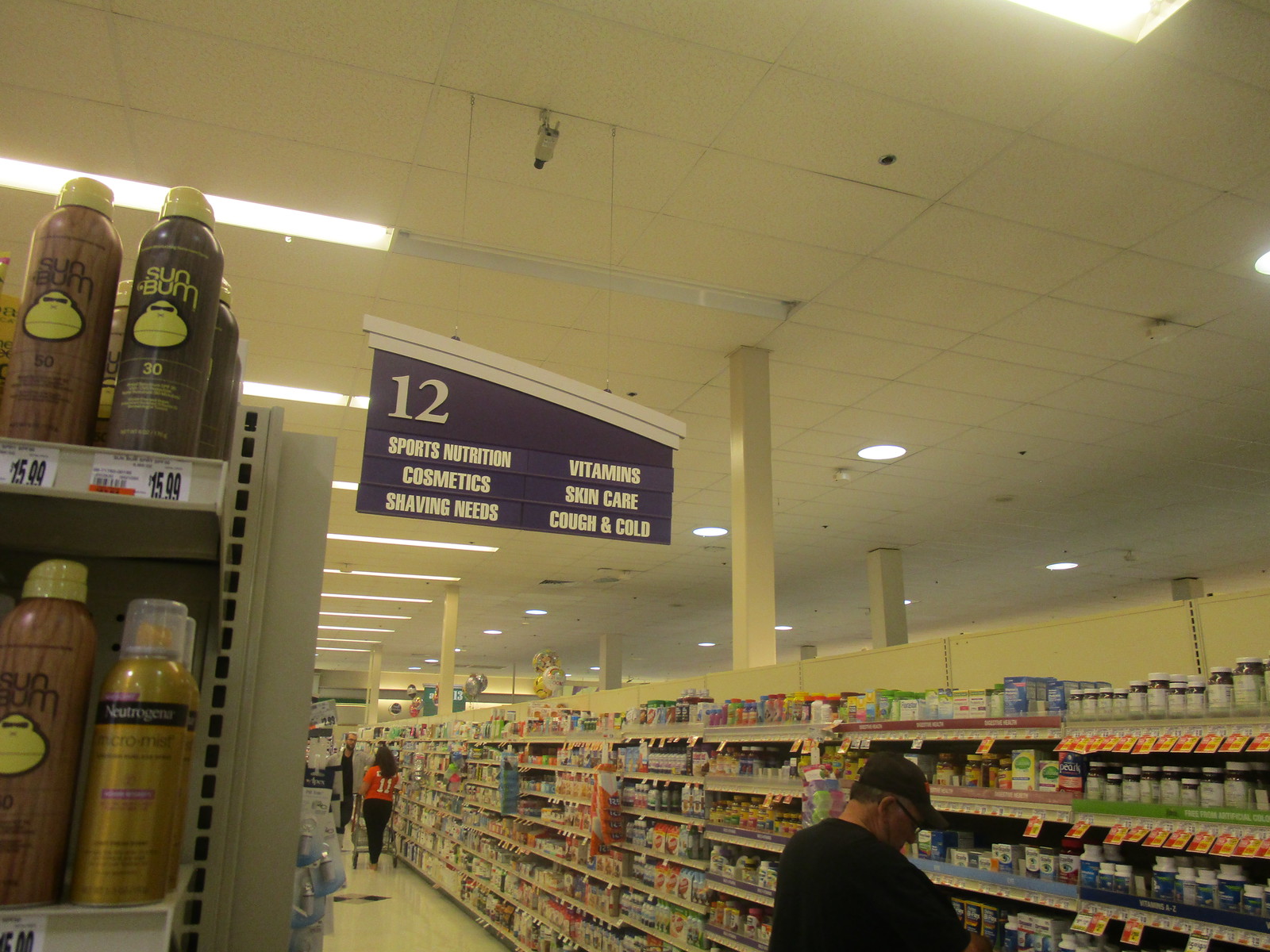The image depicts aisle 12 in a store, characterized by a white tile ceiling equipped with recessed security cameras, circular and rectangular light fixtures—one of which is not illuminated. Prominently, there is a blue sign with white text that reads: "12 Sports Nutrition, Vitamins, Cosmetics, Skin Care, Shaving Needs, Cough & Cold." The aisle stretches long, lined with relevant products. On the left, there are brown bottles with visible labels and prices, alongside recognizable brands such as Sunbum and Neutrogena. Two shoppers are visible: one is a man near the front, wearing a black t-shirt, black hat, and glasses; the other, further down the aisle, is a woman in an orange shirt and black pants engaging in conversation with a man in a white coat. The floor of the aisle is white and there are white pillars providing structural support.